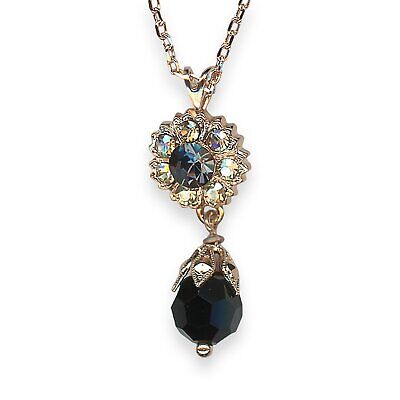The image features a detailed color photograph of a handcrafted necklace set against a white background. The necklace is composed of a gold chain link that descends to two distinct pendants. The upper pendant is circular, resembling a flower, and is encrusted with multiple cubic zirconia stones. The flower-like design of this pendant also includes a central stone that appears to be either blue or black, adding a reflective quality that contrasts with the surrounding smaller diamonds. Beneath this, another larger oblong pendant dangles, it's almost egg-shaped, and predominantly black with hints of blue. This bottom stone is adorned with a scalloped silver top, giving it a pineapple-like appearance. Together, the jewelry elements suggest a blend of gold and black tones, designed to be visually captivating without appearing overly shiny. The absence of words or additional background keeps the focus entirely on the intricate beauty of the necklace.